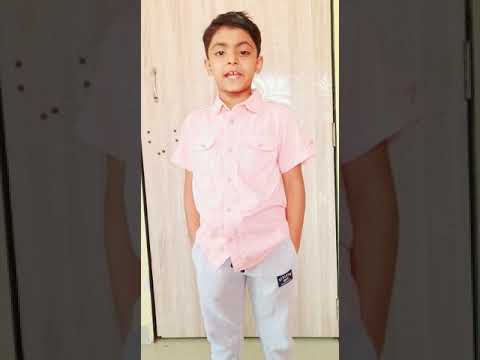This photograph captures a young boy, appearing to be about eight or nine years old, who is likely of Asian ethnicity, possibly Indian. He stands confidently in the center of the image, gazing directly into the camera with a slight smile or mid-speech expression. His dark hair is neatly cropped close at the sides, complementing his dark brows and Asian-influenced eyes. He is well-dressed, wearing a light pink button-down, short-sleeve collared shirt, paired with white trousers. Both of his arms rest at his sides, with his hands tucked into the pockets of his trousers. On the left pocket, there's a small black rectangle with white writing, likely a logo, though it's too small to discern. The interior setting features a beige-white wall and a white, slightly grayish floor. The photograph only extends to the boy's knees, leaving his footwear out of view.

Surrounding the main image are two enlarged, fragmented pictures of the boy's arms, shirt, and pants, flanking either side. These fragments emphasize the details of his attire and pose, creating a triptych effect that draws attention to his composed and engaging presence.